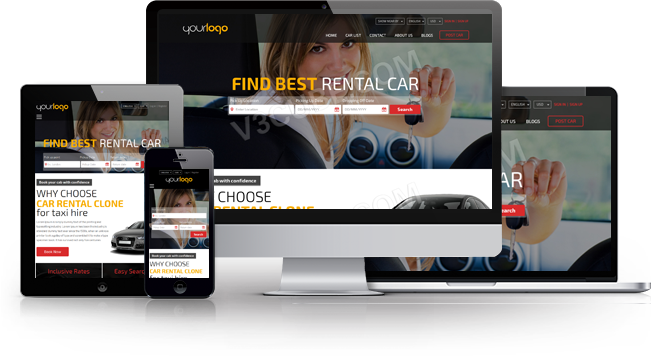This image is an advertisement showcasing a car rental website's compatibility across multiple devices. The website is displayed on four different devices: a tablet or iPad, a black cell phone, a desktop computer with a silver stand, and a laptop or Chromebook partially shown with a person's hand interacting with the screen. The central focus of the advertisement is a woman holding car keys, with a clearly visible black key and its silver tip. The promotional text at the top reads "Your Logo" and "Find Best Rental Car." Additional text promotes the service with the phrase "Why Choose Car Rental Clone for Taxi Hire," and features an image of a car alongside a noticeable red clickable button.